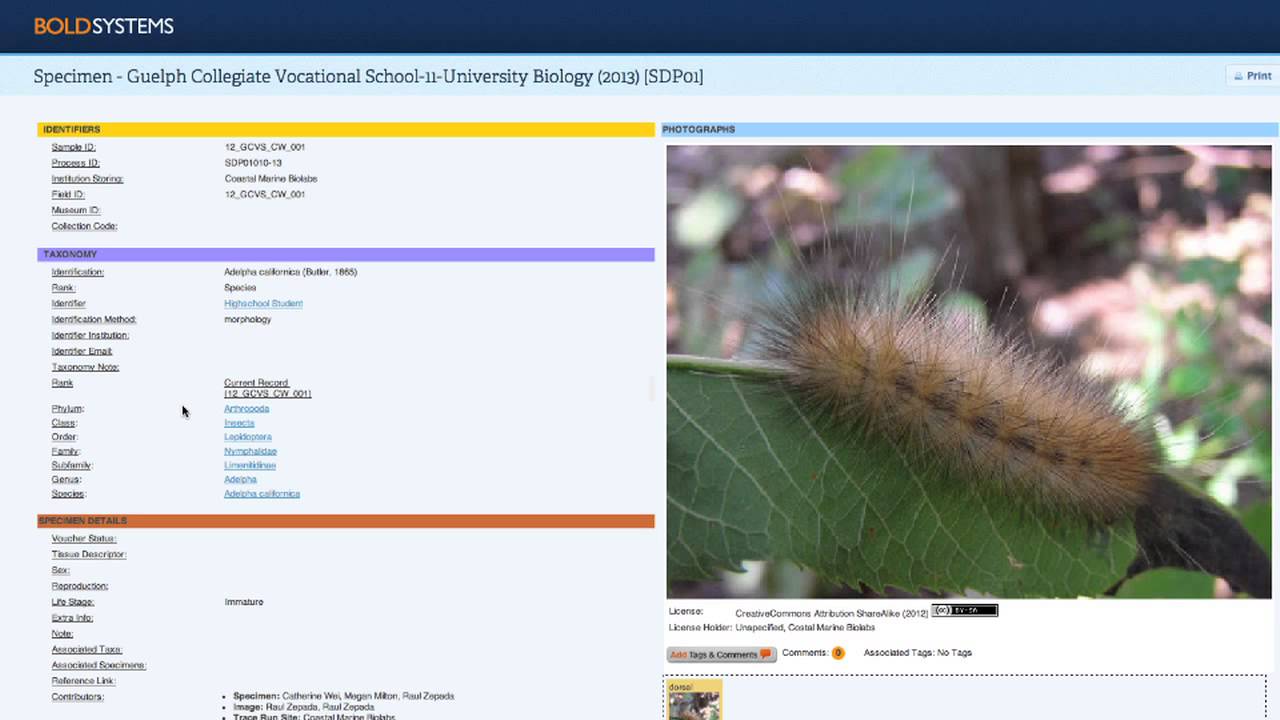### Detailed Caption:

This image shows a screenshot from a computer display featuring a well-structured, multi-colored information panel about a biological specimen. 

At the top of the screen, there is a navy banner displaying the text "BOLD SYSTEMS" with "BOLD" in orange capital letters and "SYSTEMS" in white. 

Below this, a light blue banner reads "SPECIMEN - GELF COLLEGIATE VOCATIONAL SCHOOL - 1111 UNIVERSITY BIOLOGY 2013 SDPO1."

Following this, a yellow banner with the heading "IDENTIFIERS" lists several identifiers, although some are blurry. The legible ones include:
- "MUSEUM ID"
- "COLLECTION CODE"
Next to these, it says "12GCVS-CW-001 SDPG1010-13 COASTAL MARINE BIOLABS 12GCVS-CW-001."

A violet banner beneath this, titled "TAXONOMY," appears to have clickable links which are somewhat blurry. Listed items under this banner include "IDENTIFICATION METHOD," "DISTRIBUTION," "TAXIDERMY," and "RANK." The first column contains underlined terms: "PHYLUM," "CLASS," "ORDER," "FAMILY," "SUBFAMILY," "GENUS," and "SPECIES." 

Adjacent to this column, the terms "ADELPHIA CALIFORNICA BUTLER 1865 SPECIES" and "HIGH SCHOOL STUDENT" appear in blue text, followed by:
- "MORPHOLOGY" in blue
- "CURRENT RECORD 112GCVS-CW-001" in blue
- "ARTHROPOD" in blue
- "INSECTS" in blue
- "LEPIDOSPORA METAMORPHOSIS" with some additional blurry words below.

An orange banner with the heading "SPECIMEN DETAILS" is positioned beneath these sections. It includes subheadings with black underlines such as "VOUCHER STATUS," "DESCRIPTION," "SEX," and "REPRODUCTION," though the following descriptive lines are hard to read. 

This section also includes a "NOTE" heading, followed by four more lines, one of which reads "REFERENCE LINK AND CONTRIBUTORS."

The central element of the image is a photograph of a fuzzy beige and brown caterpillar with long hairs, resting on a leaf. The background is blurred and filled with leaves. 

Below this image, the text "LICENSE CREATIVE CHAMORRES, ATTRIBUTION, SHAROQUE, 2012" is displayed, indicating the licensing details, along with "LICENSE HOLDER UNI-PACIFIC COASTAL MARINE BIOLABS." 

At the bottom, an area for user interaction includes "ADD TAGS AND COMMENTS" with a grey call-to-action button and a conversation bubble icon next to "COMMENTS, 0" in yellow, and a section marked "ASSOCIATED TAGS: NO TAGS."